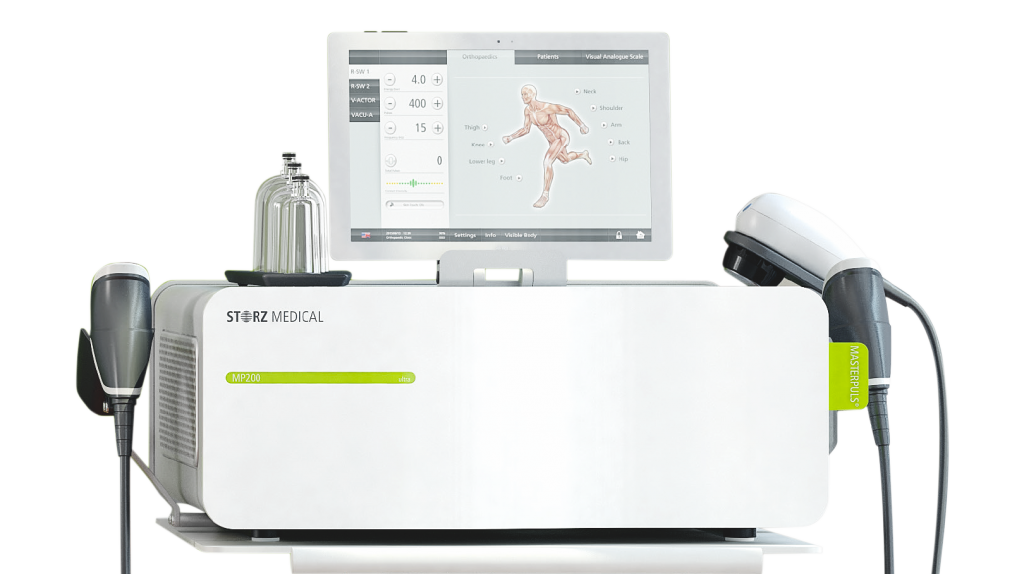The image displays a sophisticated piece of medical equipment, potentially an ultrasound or monitoring device. The machine is a large, white rectangular box resembling a computer with a prominent green bar along the side. The text "STORES MEDICAL" is printed in black letters on the upper left-hand side. There is a green line beneath this text, extending slightly longer than the lettering.

On both the left and right sides, two monitoring probes are visible, each hanging in their respective black holsters. Additionally, on the top right-hand side lies a remote control, colored in white, black, and gray. The top surface of the device houses a black tray with three clear glass bottles, each fitted with a black lid, organized from small to large.

At the center of the device, a computer screen displays various readouts, including a detailed skeletal diagram of a human body with arms extended left and right, and surrounding text providing medical data. The screen appears mounted on a bracket. The overall setup suggests a highly functional medical monitor with integrated data display and storage capabilities.